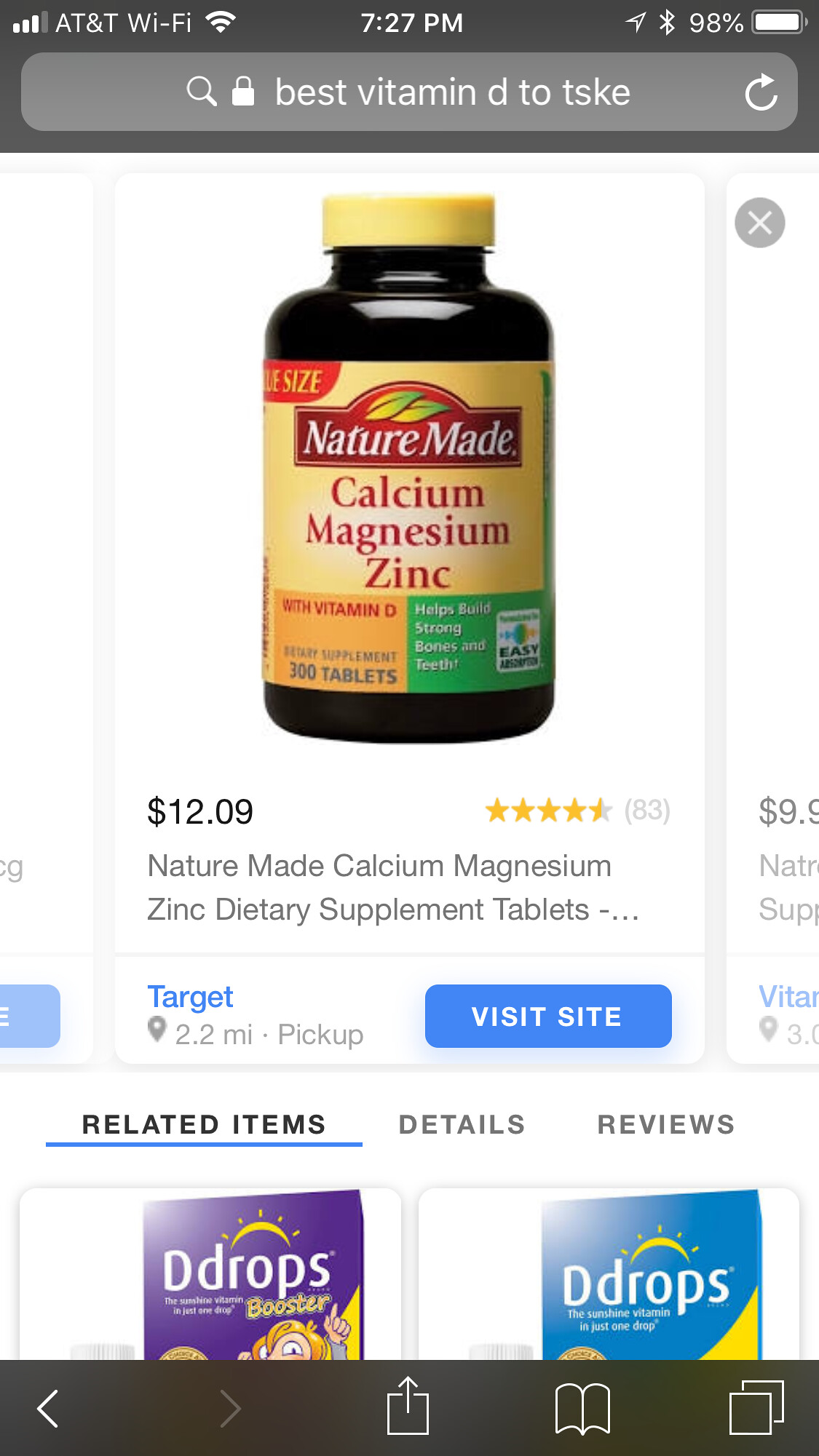This image is a screenshot taken from a smartphone, featuring a Google search for "best vitamin D to take," albeit with a typo ("TSKE"). The phone's interface displays the AT&T Wi-Fi connection on the left, along with signal strength bars. The clock in the center reads 7:27 p.m., and the battery life on the right is at 98%, with Bluetooth enabled. The search shows results featuring a Nature Made Calcium Magnesium Zinc dietary supplement. The product is displayed in a black bottle with a yellow cap and label, priced at $12.09. The listing notes it has a 4.5-star rating with 83 reviews. The advertisement includes an option to visit the Target website, indicating that the nearest Target store is 2.2 miles away. Below the main product image are related product listings, including Ddrops. The lower portion of the screen features navigation icons typical of a smartphone, including arrows and overlapping squares.